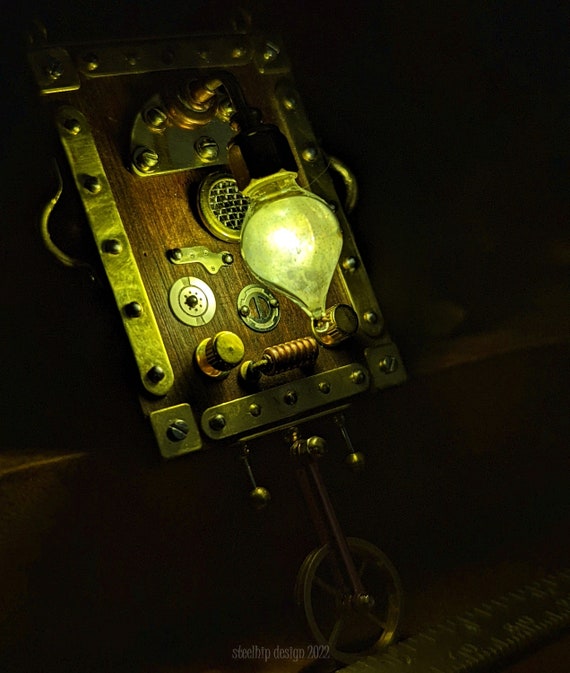The steampunk diorama showcases a detailed miniature laboratory setup centered around a rectangular, wooden board leaned against a bench or wall. This board, which has several metal rivets and screws framing it, is grey and adorned with a variety of intricate, miniaturized diagrams. These diagrams hang as pendant ornaments, circular in shape and grey in color. At the base of the board is a metallic wheel, adding to the intricate detail.

Illuminating the entire scene is a greenish-glowing glass bulb that casts a captivating light over the diorama, adding an eerie, high-tech ambiance. The overall structure resembles a part of a crate or box, secured with bolts, further indicating its robustness and mechanical complexity. This visually stunning steampunk laboratory scene, replete with high-tech gadgets and industrial decor, is reminiscent of elements one might encounter in a video game, blending the charm of antiquated technology with a futuristic twist.